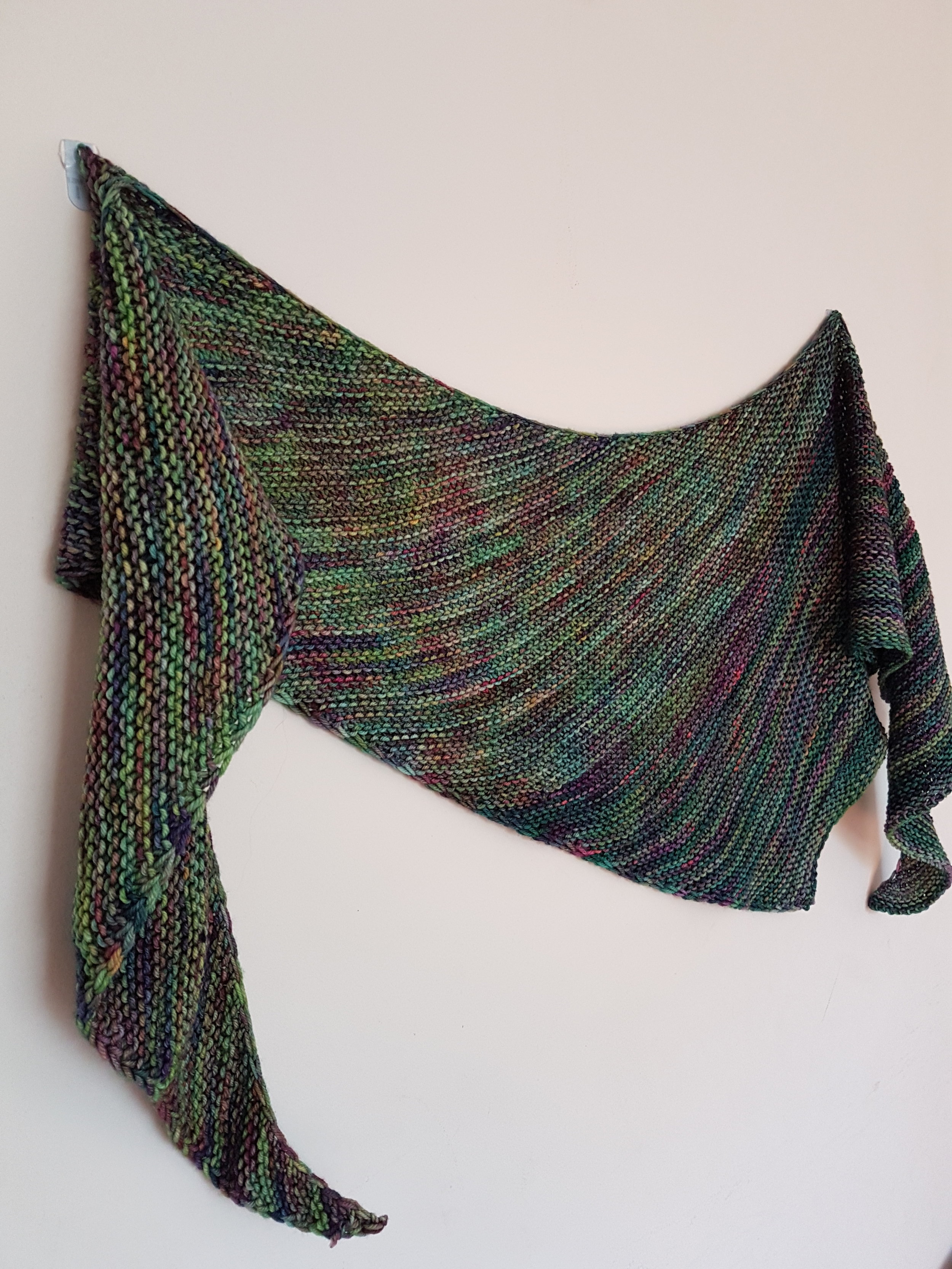The image depicts a large, shapeless piece of knitted fabric tacked to a white wall, presenting itself as an art display. The fabric features a myriad of colors, dominated by various shades of green such as olive, blue-green, and darker greens. Interspersed among these are hues of blues, patches of rusty browns, touches of red, purple, and yellow, creating a variegated effect. The overall shape could be reminiscent of a shawl or scarf, with top corners secured by white hooks, allowing the fabric to drape in a slight V-shape due to the sagging middle. The edges narrow to points and dangle below the main body of the fabric, adding to the asymmetrical, artistic appearance of the installation. The pale beige wall provides a stark, unobtrusive background, ensuring that the intricate, multicolored knitwork stands out as the focal point.